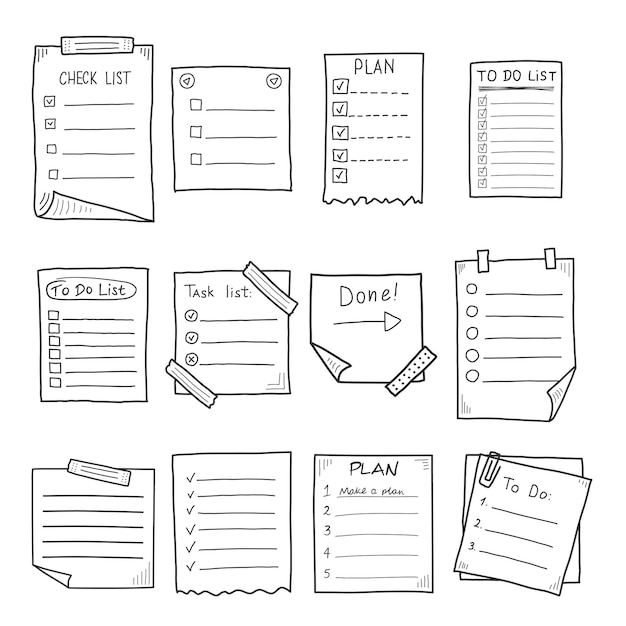The image is a collection of twelve grayscale pen-and-ink-style illustrations arranged in three rows and four columns, resembling simple, cartoon-like designs. Each illustration depicts a different type of list or document, commonly used for organizing tasks.

In the first row:
1. **Checklist on Clipboard**: A long piece of paper with the title "Checklist" at the top, displayed on a clipboard. It features several boxes beside lines, with the first two boxes checked off.
2. **Tacked Note**: A smaller square piece of paper with boxes and lines, attached by two thumbtacks at the top. Unlike the first, it lacks a "Checklist" header.
3. **Torn Plan**: Another long piece of paper, titled "Plan" at the top, with a jagged, torn bottom edge. It has checkmarks and dashed lines, with all boxes checked.
4. **To-Do List**: A list marked as "To-Do," featuring eight checkboxes, all checked, with lines next to them.

In the second row:
1. **Circled To-Do List**: A standard-sized piece of paper with "To-Do List" circled at the top. It includes about six unchecked boxes with adjacent lines.
2. **Task List with Tape**: Titled "Task List," this document features circles instead of boxes, none of which are checked. An X marks the third circle. The list is taped at the bottom left and top right corners.
3. **Sticky Note**: A small piece of paper, possibly a sticky note, titled "Done!" with an arrow pointing to the right. It has a tape piece at the bottom right corner and a folded bottom left corner.
4. **Task Circles**: Another long piece of paper with two clips or short pieces of tape at the top. It has five circles and lines, none of which are checked, with a curled bottom right corner.

In the third row:
1. **Blank Lines List**: A square piece of paper or small notepad with a clip at the top. It contains several blank lines, with the bottom left corner slightly folded.
2. **Torn List with Checkmarks**: A piece of paper torn at the bottom, displaying several checkmarks beside lines, but no specific header.
3. **Numbered Plan**: Titled "Plan," it lists items as "1. Make a Plan" followed by number two, three, four, and five, all with blank lines next to them.
4. **To-Do List with Paper Clip**: A to-do list with three items, each with lines next to them. The list is clipped at a slight angle to another piece of paper beneath it with a paper clip at the top left corner.

Each illustration portrays a different style of list, offering a variety of organizational designs, from checklists to task lists, with various methods of attachment and completion status.